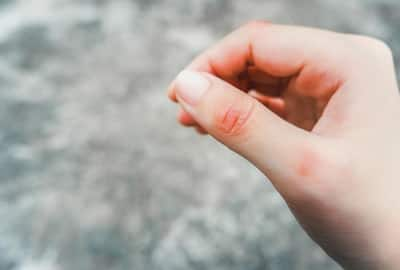This close-up photo captures a Caucasian person's hand positioned with the thumb facing the camera, creating a circle with the rest of the fingers bent to touch the thumb's tip. The background is a blend of blurred white and gray hues, providing a subtle contrast to the hand's details. The skin on the hand shows signs of irritation, particularly around the joints of the thumb, where reddish marks are visible. The redness extends slightly to the lower thumb joint and a bit beneath the fingers near the palm, suggesting possible contact with a rough surface, an injury, or a skin condition such as a rash. The image distinctly emphasizes the texture and condition of the skin, hinting at recent discomfort or irritation.